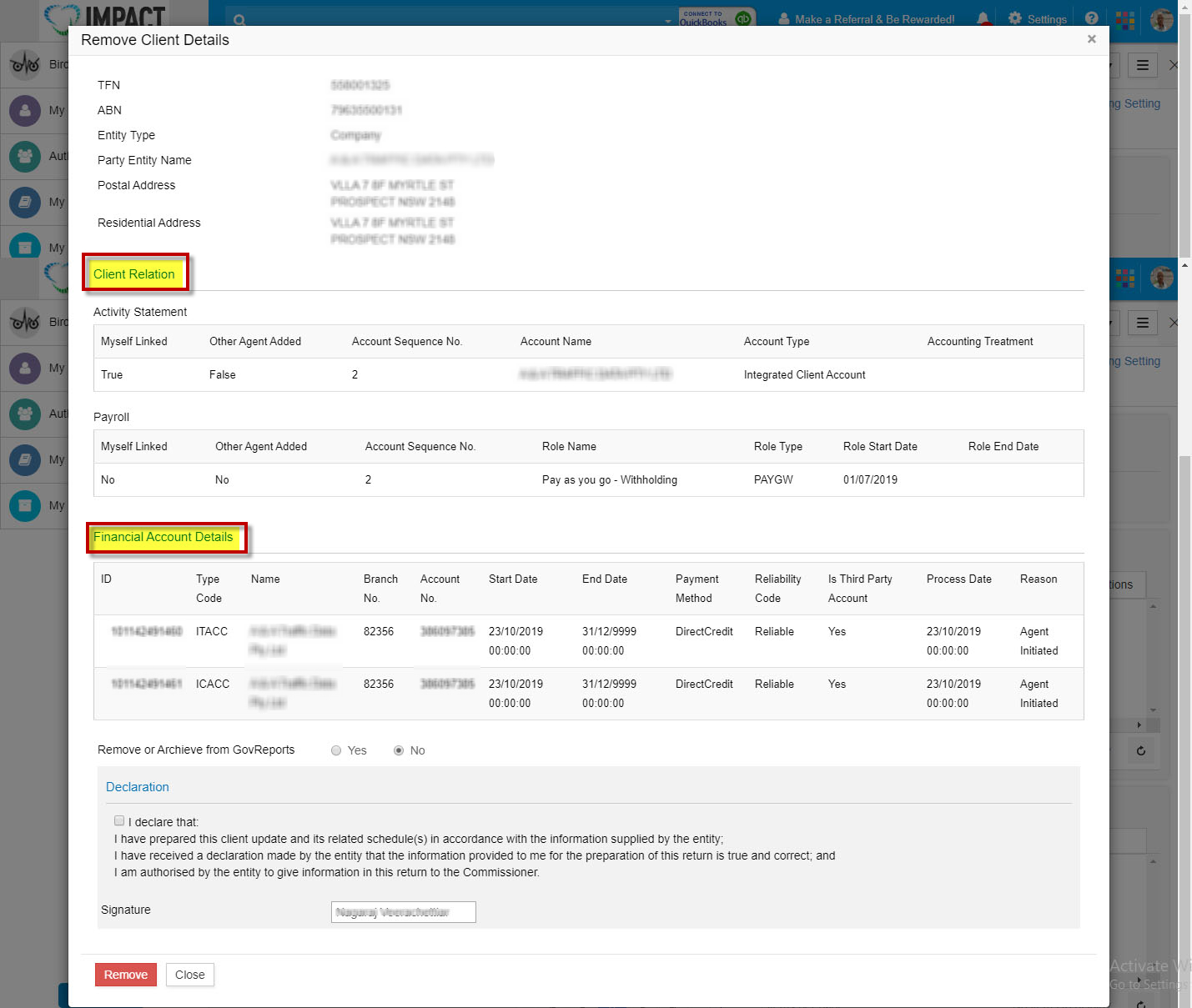This image is a detailed screenshot from a web page with most of the content obscured by a large white pop-up box dominating the central section. The underlying web page is visible only in narrow slivers on the left and right sides of the pop-up. In the upper-left corner, the partial text "impact" is discernible in a bold black font beside a cloud-shaped logo, likely representing the company's branding. The left side of the web page shows an obscured sidebar adorned with various icons.

The focal point of the image is the pop-up box titled "Remove Client Details." This section is heavily redacted, with gray blotches concealing sensitive financial information for privacy. On the left side of the pop-up, labels such as "TFN," "ABN," and "Entry Type" are discernible, while the right side features "Postal Address" and "Residential Address," with the actual details obscured.

Just below this, a yellow rectangle with a red outline displays "Client Relation," followed by another section headed "Activity Statement" against the white background. Categories listed here include "Myself Linked," "Other Agent Added," "Account Sequence," "Account Name," "Account Type," and "Accounting Treatment," again with most specific details blotted out.

Further down, another yellow rectangle marked with a red outline is titled "Financial Account Details." This part contains various categories such as "Branch Number," "Account Number," "Start Date," "End Date," "Payment Method," "Reliability Code," "Is This Third Party Account," "Process Date," and "Reason," all of which are redacted.

At the image's very bottom, in blue font, the word "Declaration" is visible along with text stating, "I declare that I have prepared the client update," indicating a required affirmation of the accuracy and validity of the provided information, though the full content of the declaration is partially unreadable.